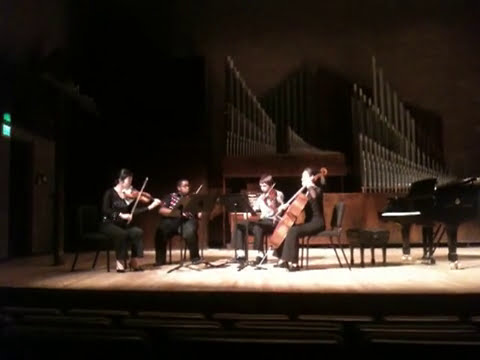The image depicts a classical string quartet in the midst of performing a musical piece on stage. Four musicians—three violinists and one cellist—are positioned centrally, all attired in black outfits and seated on black office-style chairs. In front of each musician, there are music stands that hold their sheet music. The stage is adorned with a light brown hardwood floor, which extends beneath their feet. 

To the right of the musicians, a grand black piano with white keys stands prominently, accompanied by a piano bench. Further in the background on the right side, there is a majestic dark brown organ, its silver pipes reaching upwards, reminiscent of those found in grand churches. The scene suggests a practice session or live performance, capturing the elegance and seriousness of a classical music setting.

Adding a touch of visual contrast, an aqua-colored light emanates from a small window or fixture located in the left corner of the image. The overall composition is rich in detail, highlighting the juxtaposition of the wooden floors, dark brown organ, and sleek black piano against the musicians' focused expressions and practiced movements.